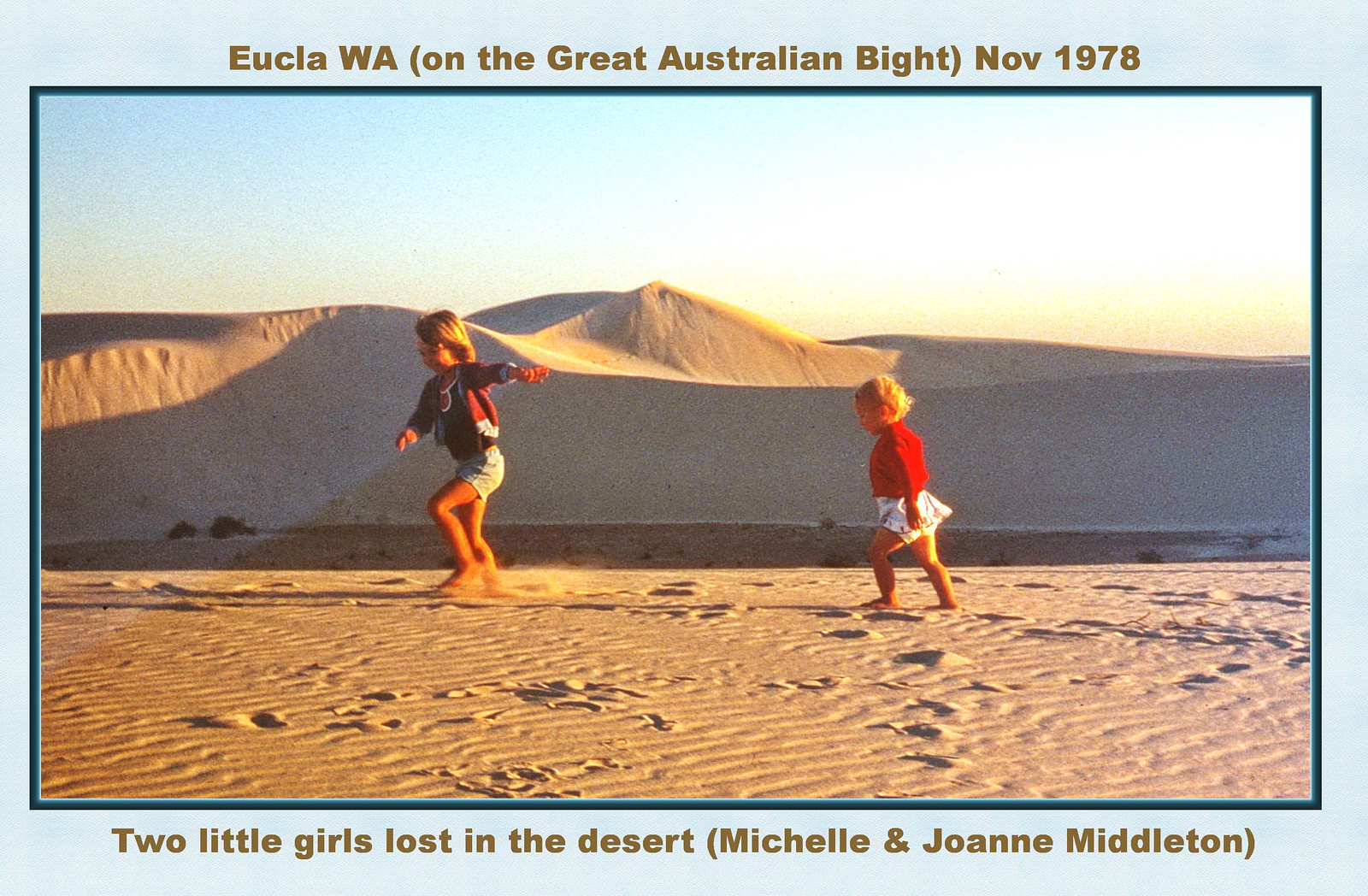In the photograph, taken in November 1978, two small barefoot children are seen walking on a sandy, flat surface of a desert near Eucla, WA, on the Great Australian Bight (spelled B-I-G-H-T). The text above the image, placed in parentheses, reads "E-U-C-L-A, capital W, capital A, on the Great Australian Bight," while the caption below states, "Two little girls lost in the desert, Michelle and Joanne Middleton." The older child, possibly around five years old, who has short blonde hair, is on the left. She is wearing a light jacket with shorts. The younger child, a toddler likely still in diapers, is on the right. She is clad in a red top and a white skirt, also with blonde hair. The children are making footprints in the sand as they seem to be moving forward toward the left. In the background, a large sand dune rises against a visible sky occupying the upper third of the image. The picture is bordered in light blue, and the text is inscribed in gold against a lighter blue background.